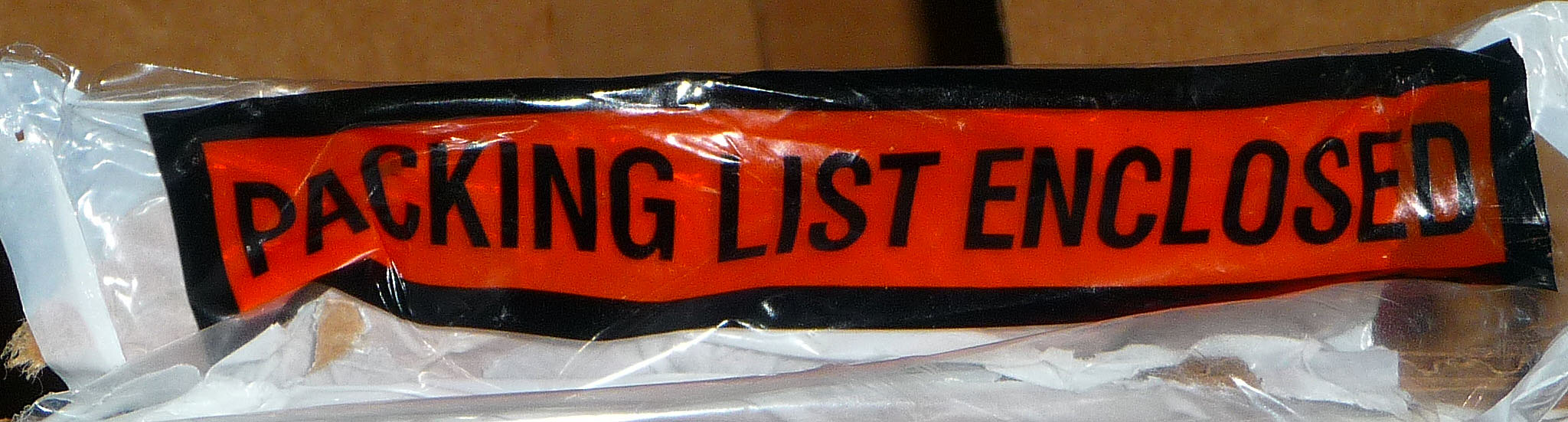The detailed photograph is a close-up of a small, rectangular, oblong-shaped plastic packet with a transparent front and a white background. The packet prominently features the text "PACKING LIST ENCLOSED" in capital letters, printed in black. This text is encased within a red rectangle, which in turn is bordered by black. The photograph is brightly lit, clearly showing the type and details of the packaging. The packet appears to be lying on a brown surface, possibly a table or countertop. There are no people, furniture, cars, or any other elements in the image—just the focused shot of the package itself.